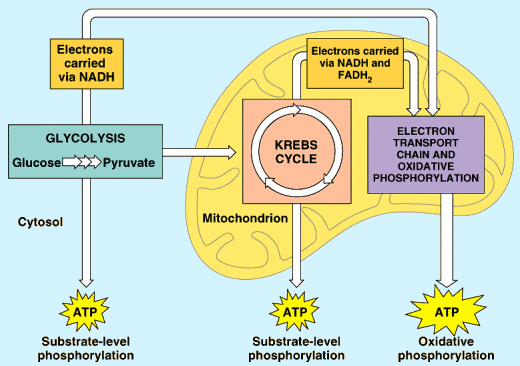This detailed diagram illustrates the Krebs Cycle within the brain, emphasizing the metabolic pathways and energy production processes. The central focus is a large, kidney-shaped yellow outline representing the mitochondrion, situated on the right-hand side of the image. This shape contains multiple interconnected arrows and boxes detailing the steps of the Krebs Cycle.

Key features include:

- **Upper Left Corner:** A rectangular box labeled "electrons carried via NADH" against a light blue background, initiating the flowchart.
- **Pathways to the Right:** From this box, arrows lead to additional stages including glycolysis, glucose, and pyruvate, eventually connecting to a yellow lightning icon labeled "ATP" and "substrate-level phosphorylation."
- **Lower Left Corner:** An orange and a blue box, each also connected to ATP bubbles via arrows.
- **Curved Oval Shape (Right Section):** Inside the mitochondrion, numerous rectangles contain specific details such as the Krebs Cycle, electron transport chain, and oxidative phosphorylation. These elements are visually connected by a series of arrows and pathways.
- **Brain Illustration:** Positioned on the right-hand side, a detailed brain graphic features three colored boxes (orange, pink, purple) with arrows extending toward cartoon-like chat bubbles labeled "ATP."
- **Additional Details:** Throughout the diagram, repeated terms like electrons carried via NADH, glycolysis, ADP, and oxidative phosphorylation are prominently noted, illustrating the complex interplay between these biochemical processes.

Overall, the background color is light blue, providing contrast and clarity to the intricate relationships depicted in this scientific flowchart.